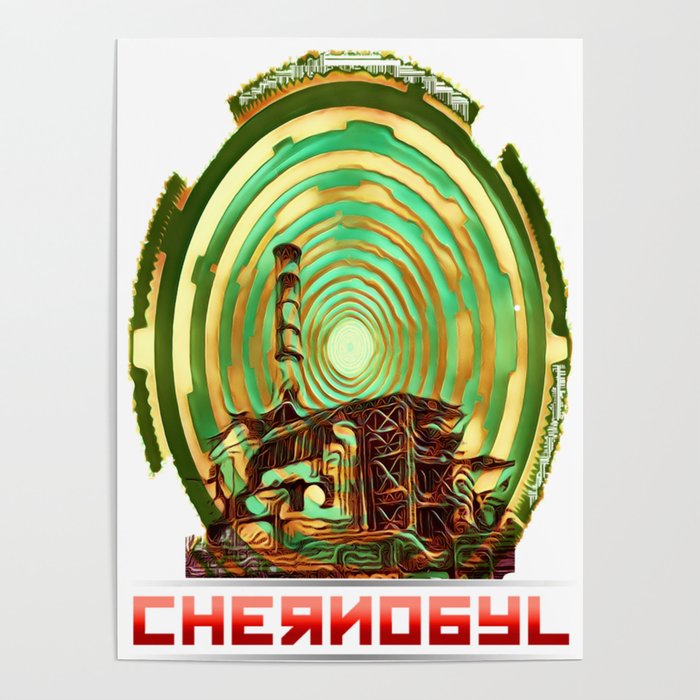The image is a vertically rectangular colored print piece with a light gray border, thicker on the left and right than on the bottom. Inside, against an off-white background, there is an abstract graphic depicting a factory-like building with a smokestack on the left, seemingly melting. Above the building, green and gold concentric circles with wiggly edges create a surreal effect, possibly representing radiation or energy waves. At the bottom of the image, in large bold capital letters, "CHERNOBYL" is spelled in red with a gradient from pink at the top to dark red at the bottom, and the 'R' is reversed, adding to the disorienting and abstract nature of the piece. The overall composition conveys a sense of distortion and decay, evocative of the Chernobyl disaster.